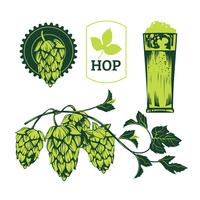The image is a detailed logo for a beer company, heavily emphasizing the use of hops in brewing. Central to the design is a green emblem featuring a thin outline and three leaves, with the word "hop" prominently displayed beneath in dark green text. To the left of the central emblem, there's a gear-shaped circle containing a downward-facing hop illustration. On the right side, the image showcases a tall, green-shaded beer glass with visible foam at the top. The background is predominantly white, creating a striking contrast with the varying shades of green. Below these elements, a horizontal vine stretches across the width of the logo, adorned with four hanging hops. The overall design intricately combines various hop and beer imagery to represent the brewing process.